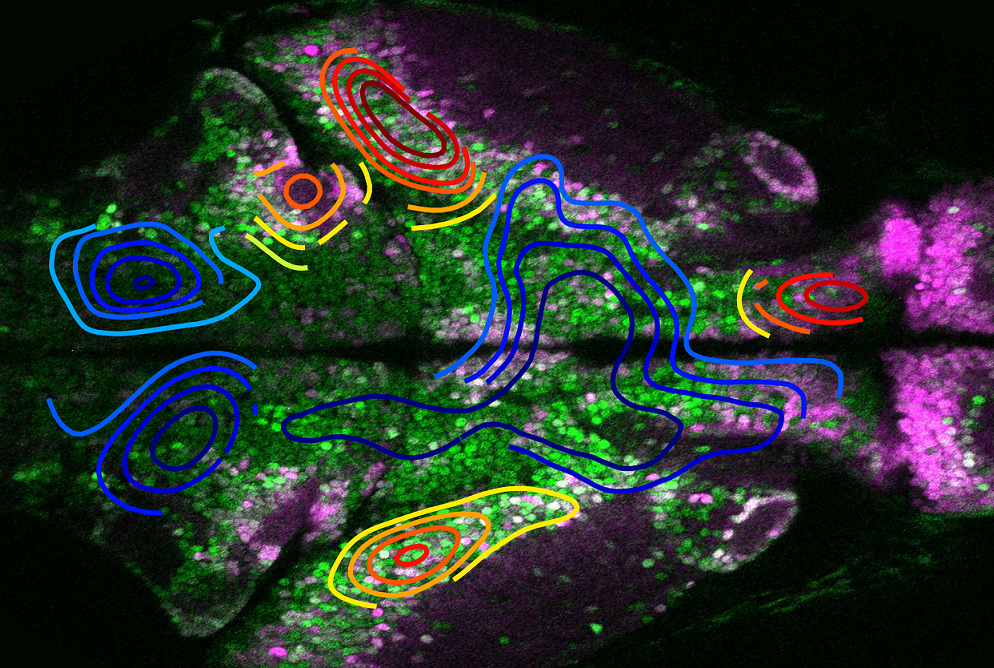The image showcases a vibrant, kaleidoscopic array of colors and patterns against a black background. Fluorescent dots in shades of green and purple, arranged in geometric forms, seem to coalesce towards the center and disperse towards the edges. The left side of the image mirrors the right, creating a symmetrical split down the middle. Overlaid on this colorful backdrop are thick, spiraling lines and swirls in bright fluorescent blue, yellow, orange, and red hues. These drawn shapes form intricate circular patterns and long, squiggly lines, reminiscent of someone using a fluorescent pen to doodle over a kaleidoscope-like design. The entire composition is speckled with glittery particles, adding to the overall dazzling effect.